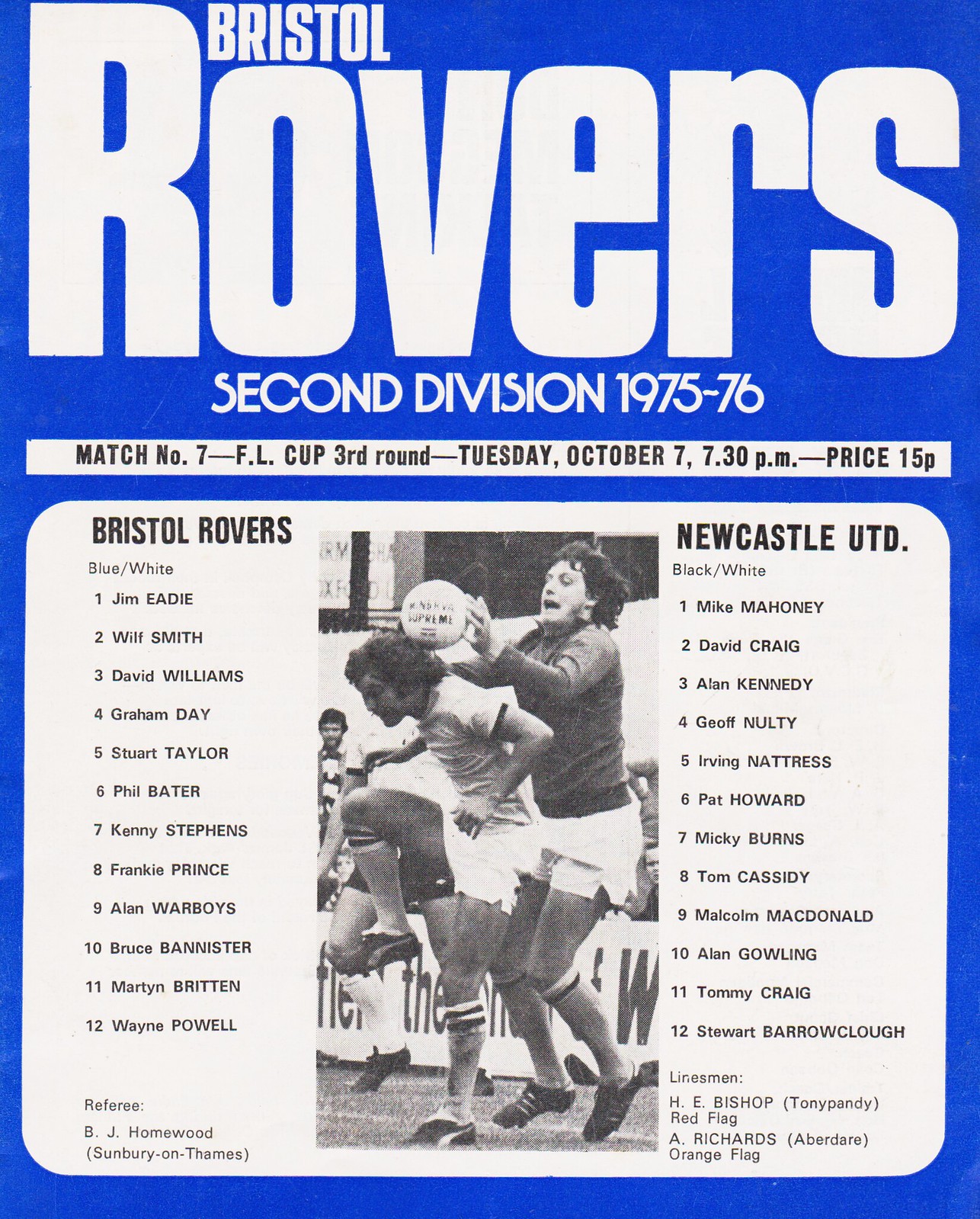The image appears to be a magazine cover or newspaper insert for a soccer match. The cover features a predominantly blue background with white and black text. At the top left corner, in white text, is the title "Bristol." Below and across a significant portion of the page is the word "Rovers" in large white font, with the smaller text "2nd Division 1975-76" beneath it. Further down, a white rectangular box with black text reads: "Match No. 7 - F.L Cup 3rd Round - Tuesday, October 7, 7.30pm - Price 15p." 

In the center, there is a black-and-white photograph depicting two soccer players in action; the player on the left wears a white uniform, while the player on the right sports a black shirt with white shorts. Below this image, another white box lists the teams. On the left side, under "Bristol Rovers blue/white," the names listed are: Jim Eadie, Will Smith, David Williams, Graham Day, Stuart Taylor, Bill Bater, Kenny Stephens, Frankie Prince, Alan Warboys, Bruce Bannister, Martin Patching, and Wayne Powell. On the right side, under "Newcastle UTD black/white," the names listed are: Mike Mahoney, David Craig, Alan Kennedy, Jeff Nolte, Irving Nattrass, Pat Howard, Mickey Burns, Tommy Cassidy, Malcolm Macdonald, Alan Gowling, Tommy Craig, and Stuart Barrowclough.

At the bottom, the officials are named in black text on a white background: referee B.J. Homewood from Salisbury, with linesmen H.E. Bishop and Tony Panty (red flag) from Redruth, and A. Richards (orange flag) from Aberdare.